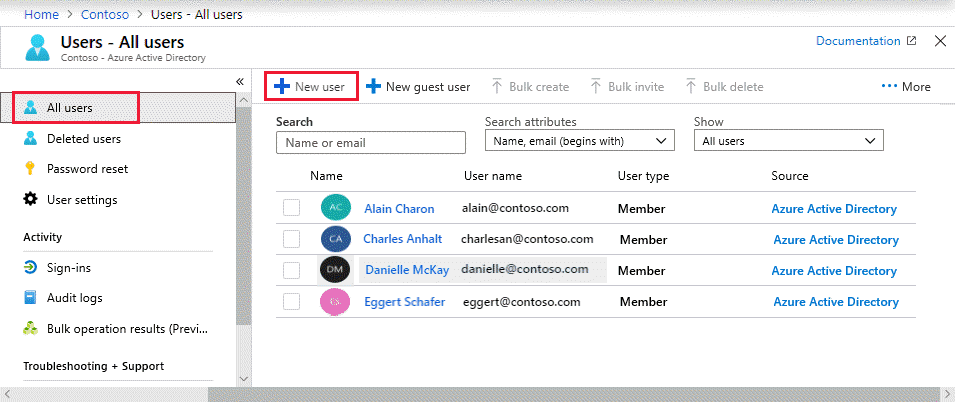In this image, the interface of the Contoso Azure Active Directory dashboard is displayed. At the top left corner, there are navigation breadcrumbs indicating the user's path: "Home" followed by a right arrow, "Contoso" with another right arrow, leading to "Users" and then "All Users." The words "Home" and "Contoso" are highlighted in light blue, while "Users" and "All Users" are bolded in black text.

Continuing below, the text "Contoso Azure Active Directory" appears in smaller font size. On the far left middle section of the page, there is a list of categories: "All Users," which is highlighted with a red rectangle around it, followed by "Deleted Users," "Password Reset," and "User Settings." Another section labeled "Activity" follows, distinguished by bold black text and a thin horizontal line beneath it, separating it from the categories above. Under "Activity," the options listed are "Sign-ins," "Audit Logs," and "Bulk Operation Results."

Towards the top center, slightly to the left, the option "New User" is displayed inside a red rectangle, accompanied by a blue plus button. To its right, there is the option "New Guest User," also with a blue plus button to its left. Directly below these buttons, there are three text boxes. The first text box is labeled "Search" with the placeholder text "Name" inside it, the second box labeled "Search Attributes," and the third box labeled "Show."